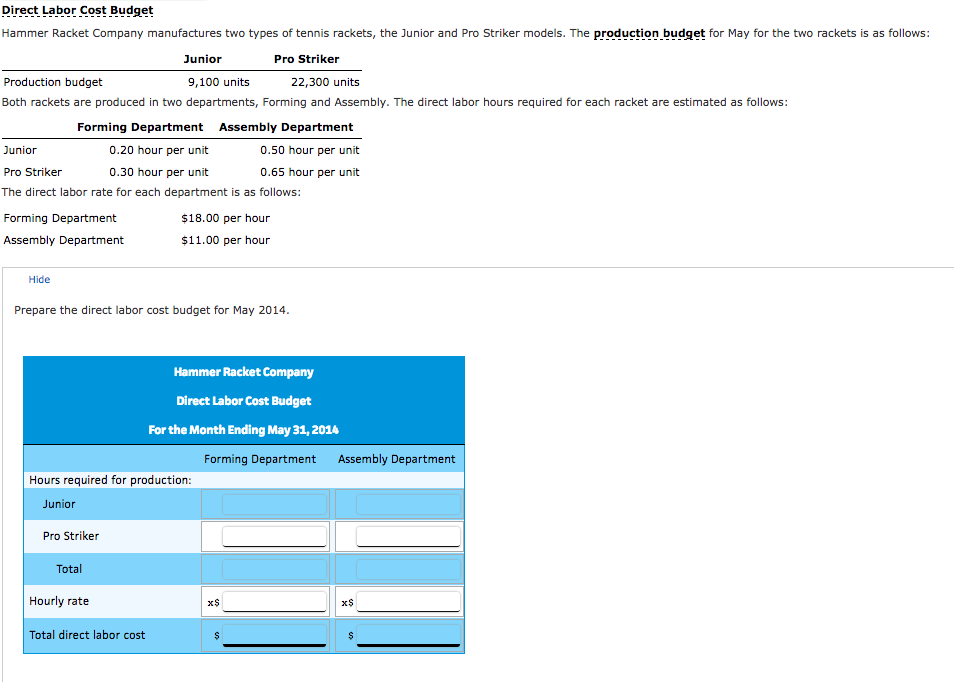A detailed screenshot displays a labor cost budget for Hammer Racket Company, specifically designed for the month of May. The image has a plain white background, emphasizing its focus on the information presented.

The title "Direct Labor Cost Budget" is prominently displayed at the top, underlined by a dotted line. Below the title, a brief explanation details that Hammer Racket Company manufactures two models of tennis rackets: the Junior and the Pro-Striker. This section notes that the production budget for May is highlighted, with the terms 'Production Budget' bolded and underlined, suggesting potential hyperlinks.

A well-organized table presents the production budget, listing 9,100 units for the Junior model and 2,300 units for the Pro-Striker model. It further elaborates that both rackets are manufactured in two departments: Forming and Assembly. Another table outlines the estimated direct labor hours required per racket and provides the labor costs. The Forming Department’s labor rate is specified at $18 per hour, while the Assembly Department's rate stands at $11 per hour.

At the bottom of the screenshot, there is a user-interactive table where custom values can be inputted to compile the direct labor cost budget for May 2014. This feature indicates that the screenshot likely comes from an older bookkeeping program, considering the reference to a date ten years prior.

Overall, the image provides a comprehensive breakdown of labor costs associated with the production of two tennis racket models at Hammer Racket Company, complete with sections for user input and detailed cost analysis.